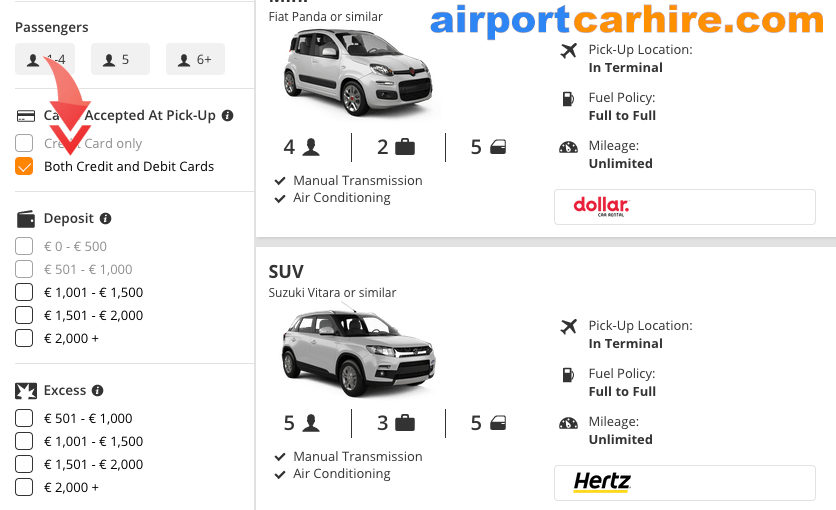**Screenshot Description of AirportCarHire.com Website:**

This screenshot depicts the AirportCarHire.com website, showcasing car rental options for passengers arriving at the airport. On the far left, there are filtering options for the number of passengers: 1-4, 5, and 6 or more. Below this, a red arrow points downward highlighting that both credit and debit cards are accepted. Further down, there are filters for deposit ranges (£0-£500, £501-£1,000, £1,001-£1,500, £1,501-£2,000, and £2,000+), and none are selected. Similarly, there are filters for excess amounts (£501, £1,000, £1,001-£1,500, £1,501-£2,000, and £2,000+), all of which are unchecked.

To the right of these filters, set against a white background, is the main content area of the website featuring the AirportCarHire.com logo. Below the logo, there is a listing for a car rental option: a Fiat Panda (or similar) with an image of a white car. This vehicle accommodates 4 passengers, has space for 2 briefcases, features 5 doors, and comes with a manual transmission and air conditioning. Additional details include the pickup location at the terminal, a full-to-full fuel policy, and unlimited mileage. This option is available from Dollar Car Rentals.

Below, there is another car rental listing for an SUV, specifically a Suzuki Vitara (or similar). This SUV can hold 5 passengers with 3 rows of seats, has 5 doors, and also features a manual transmission and air conditioning. Similar to the Fiat Panda, pickup is at the terminal, with a full-to-full fuel policy and unlimited mileage. This vehicle is available for rent from Hertz.

This screenshot effectively displays the available car rental options at the airport for immediate collection upon arrival.